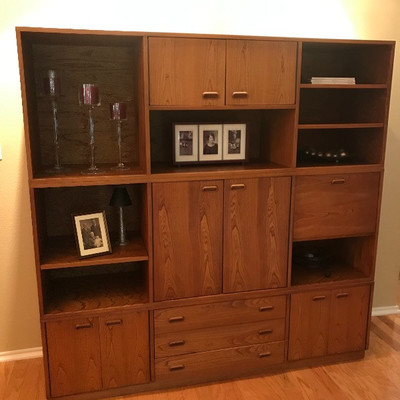This image depicts a large wooden cabinet, possibly made of wood or laminate, situated against a greenish-yellow wall with a bright light source that may be an LED strip light at the top of the cabinet. The structure appears to be an entertainment center without a section for a TV, consisting of a series of drawers, doors, and open shelves arranged in a functional layout.

On the left side of the cabinet, there are three open shelves, the uppermost of which contains three tall glasses arranged in descending height from left to right. Below this shelf, the next compartment holds a framed picture and a small lamp, followed by an empty space and a pair of small doors at the bottom.

The central part of the cabinet features a pair of medium-sized cabinet doors at the top, with a single shelf below it displaying three framed pictures. Beneath this is a larger cabinet with two doors, followed by three long drawers at the base.

On the right side, there are several open shelves at the top, one of which contains various unidentified items, possibly including a book. Additionally, there is a cabinet with a single door and a shelf. The bottom part of the right side includes two small doors.

The entire structure stands on a hardwood or laminate floor, and it has a cohesive wooden texture, adding to its aesthetic appeal.